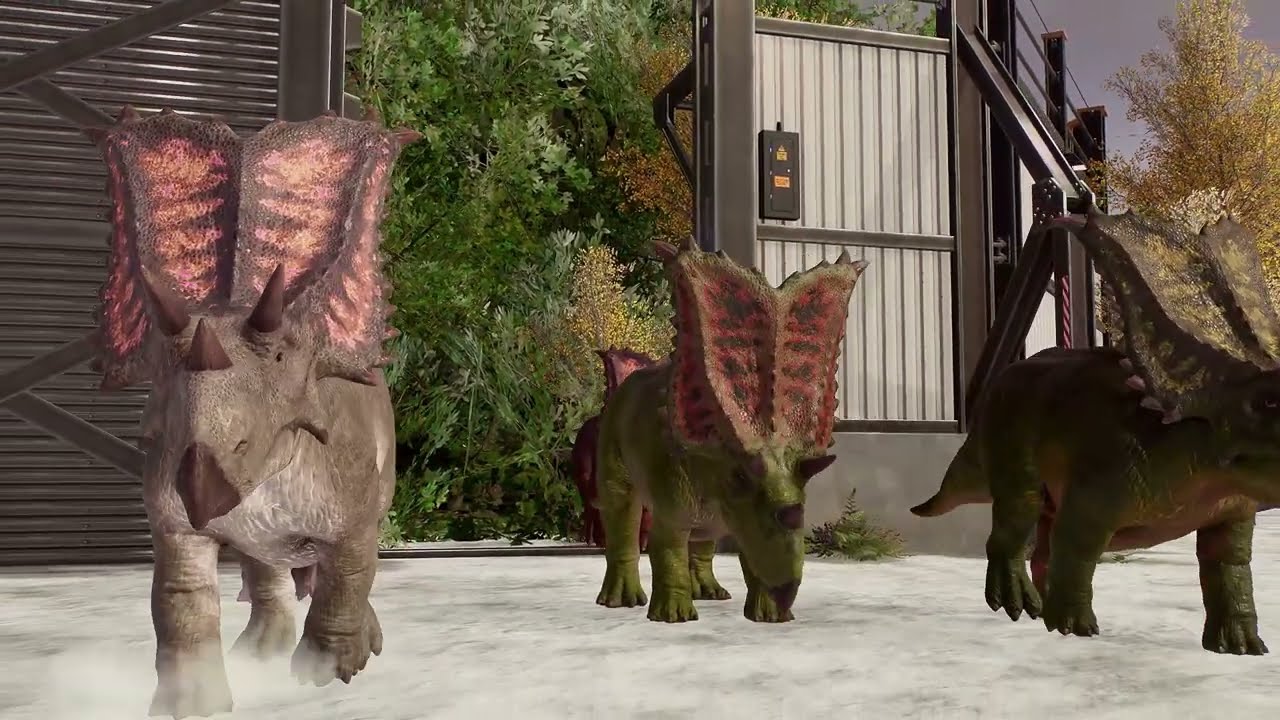The digitally rendered image vividly depicts a natural outdoor setting, seemingly taken from a video game with a Jurassic Park theme. The scene features a trio of triceratops dinosaurs prominently positioned in the center, roaming on a snow-covered ground. The triceratops display a variety of colors; some have green bodies, others gray, while their distinctive head shields exhibit shades of reddish hues. 

Encircling the dinosaurs is a walled area constructed from corrugated steel and supported by brown steel girders. The wall is topped with barbed wire, reinforcing the enclosure's purpose. To the left of the scene, there is a sturdy gray fence, while directly behind the triceratops stands a structure resembling a storage shed, made even more intriguing by its window with white shades that could be mistaken for a remote control box. 

The dinosaurs are depicted as having three horns: two above their eyes and one on their nose, with ears that slightly resemble butterfly wings. Surrounded by lush trees with green leaves, the setting suggests a secure but open outdoor area still protected from the outside world, evoking the sense of a lush, prehistoric preserve. The entire scene is meticulously detailed, showcasing the vivid colors and lifelike textures typical of high-quality digital rendering.